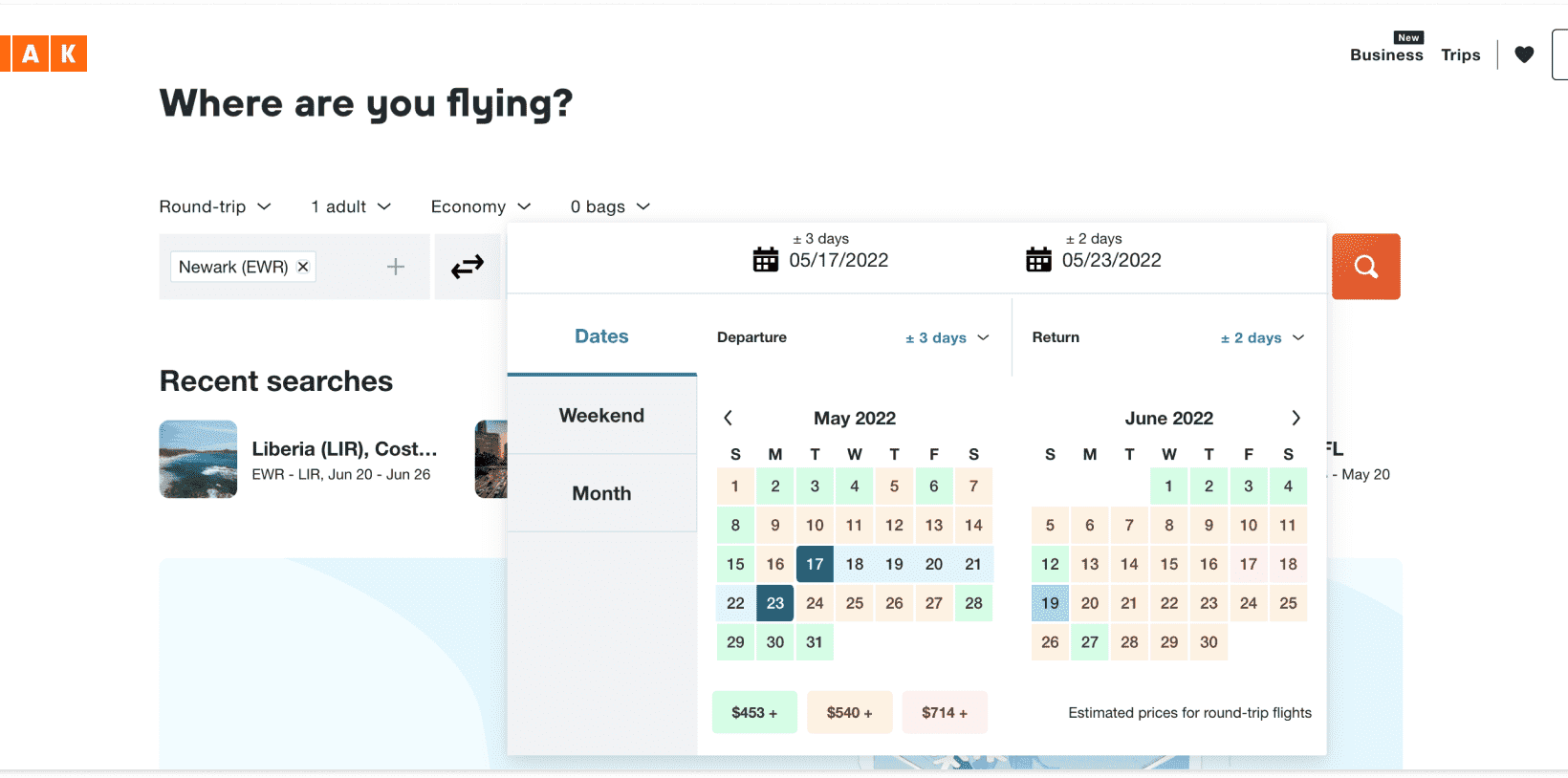**Detailed Caption:**

The screenshot, taken in landscape mode likely from a laptop, predominantly features a white background with various interface elements superimposed. At the top, spanning from the upper left to the upper right, is a white navigation bar. On the upper left, an orange square displays the letters "A" and "K." The upper right section lists options labeled "Business" with a "New" rectangle icon, "Trips," and a heart symbol indicating favorited items. Centered below the navigation bar is a bold prompt, "Where are you flying?"

The next row contains header tags, including "Round Trip" with a dropdown arrow, "1 Adult" with a dropdown arrow, "Economy" with a dropdown arrow, and "0 Bags" with a dropdown arrow. Following that, on the leftmost column, a gray label indicates the departure airport "Newark, EWR" next to a dismiss option (X). Adjacent to it, a double arrow symbol signifies a round-trip flight.

Further down in the first column, a bold section titled "Recent Searches" lists a previous search for flights from "EWR to Liberia" (coded as LIR) with the dates June 20th to June 26th. This section is flanked by small images on either side.

A pop-up calendar menu overlays the bottom part of the screen. The top row of this section displays date ranges indicating May 17th, 2020, to May 23rd, 2020, with a flexible option of plus or minus two days. To the right, an orange search bar is situated alongside three main columns labeled "Dates," "Departure," and "Return," each showing distinct calendar dates. The bottom strip of the image transitions from light blue to blue, providing a subtle separation from the rest of the interface.